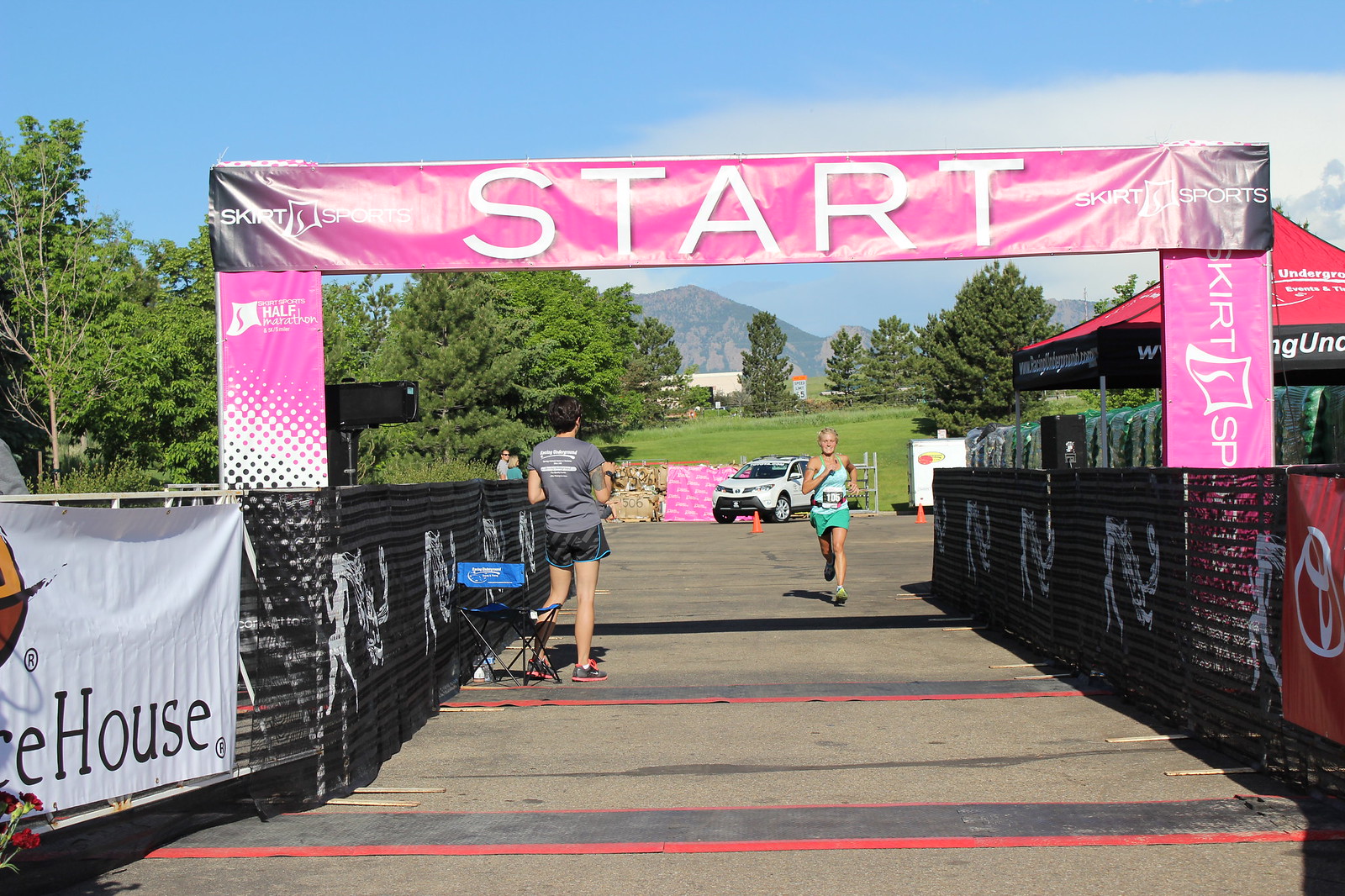A vibrant photograph captures what appears to be the finish line of a running race. Dominating the scene is a pink, black, and white archway centered in the middle of the image, symbolizing the end of the race. Just off-center to the right, a woman is captured mid-stride, seemingly close to finishing her race as there are no other runners in sight. This lone runner is being cheered on by another person positioned to the left, beneath whom a small chair is visible. Below the archway, on both sides, stand black, white, and red barriers marking the race course.

In the background, a white car is following the runner, a common practice to ensure the safety of the race participants. The landscape behind them features light green trees and a distant mountain painted in brown and green hues. Topping off the scenery, the sky stretches across the top third of the image in a serene light blue.

Text elements are subtly included in the image, with the words "start," "skirt," "sports," and "house" visible, adding an extra layer of context. The overall scene brims with a sense of triumph and conclusion, highlighting the determined runner and the supportive atmosphere at this race's end.